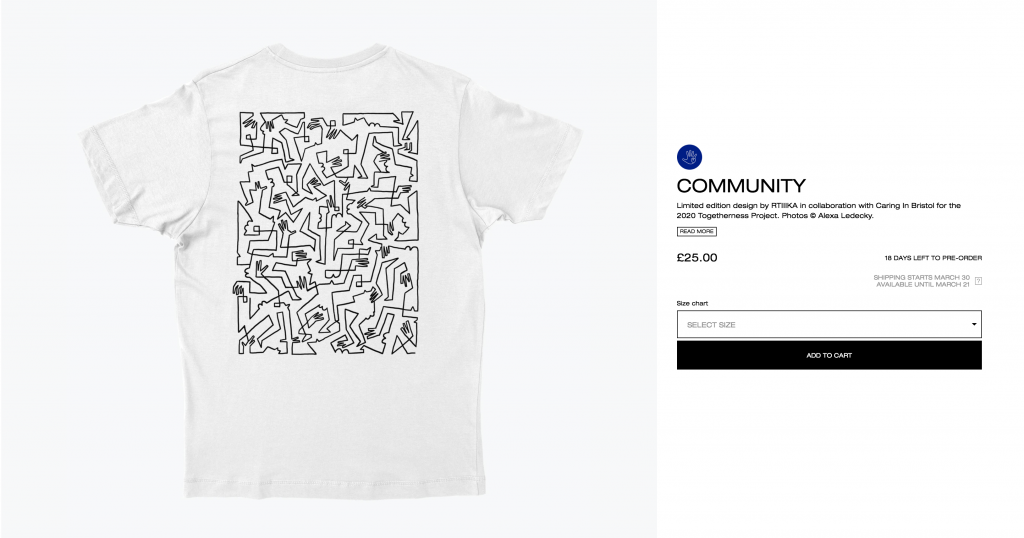This image features a webpage from an online clothing store displaying a featured product. The focal point is a white T-shirt adorned with a black design, placed against a pristine white background. On the right side of the T-shirt, there is detailed product information. 

A notable blue icon, depicting a hand, is labeled "Community." Below this icon, there is a description stating, "Limited edition design by R. Tika in collaboration with Caring in Bristol for the 2020 Togetherness project. Photos by Alexa Ledki." There is a "Read More" link to the left of this description.

The price of the item is listed as €25, with a note indicating that there are "18 days left to pre-order." Further details highlight that shipping will commence on March 30th, and the item will be available for purchase until March 21st. 

Below this information, a small "Size Chart" link appears on the left, followed by a sizable bar for selecting the desired size. At the bottom, a prominent black button reads "Add to Cart."